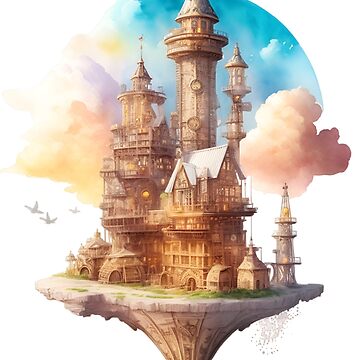The image is a detailed artistic rendering, possibly a watercolor or digital painting, showcasing a futuristic castle set atop a floating, circular island. The island features tall pillars and columns, with a large, multi-towered structure made up of light brown buildings and huts, some topped with white roofs and surrounded by patches of green grass. The floating island comes to a point at the bottom and is set against a sky filled with vibrant, colorful clouds that transition from pink and orange to yellow and purple tones. A solid blue half-circle arcs behind the scene, adding a touch of surrealism. Despite the daytime setting, subtle illumination highlights the structure, casting a slight yellow glow. Three gray-outlined birds are seen flying to the left of the composition, linking the serene, sky-bound environment.